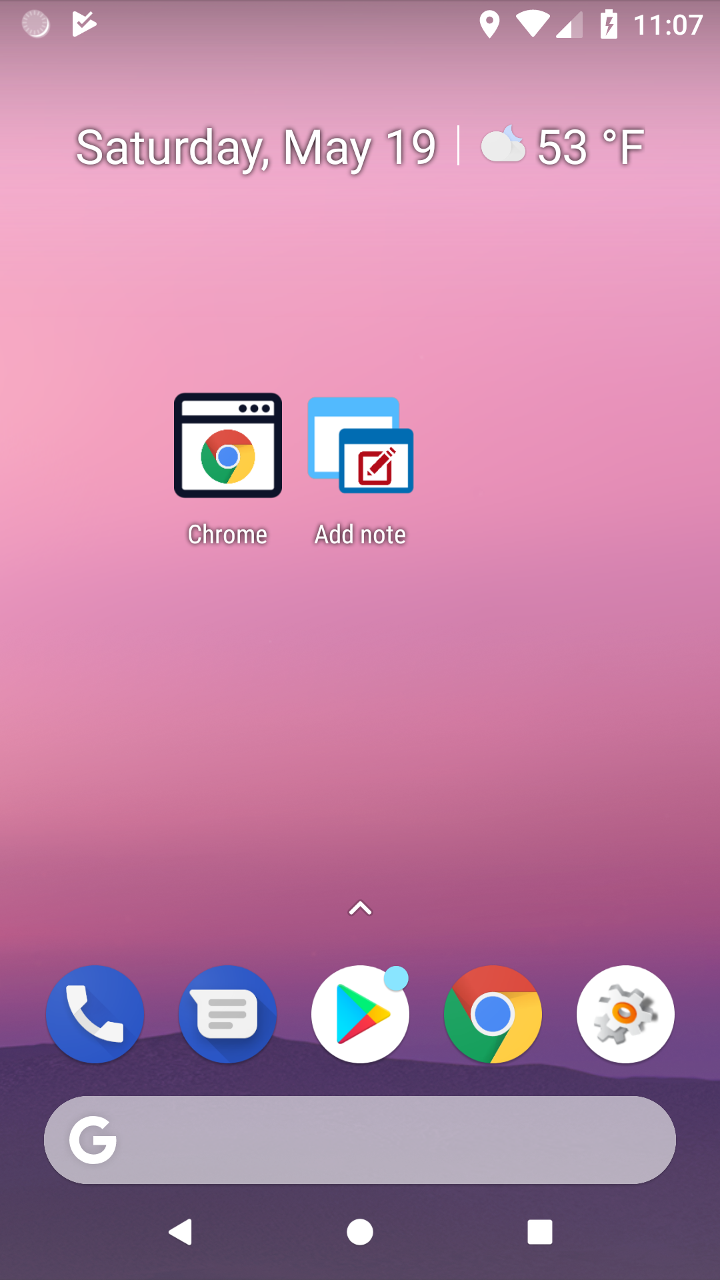The screenshot appears to be from a smartphone’s home screen, featuring a visually appealing background with a gradient ombre that transitions from lilac to pink and back to lilac before ending in a deep purple hue. A minimalist mountain silhouette in purple contrasts beautifully against the pink background at the very bottom.

At the top of the screen is a circular icon along with a tilted triangle containing a checkmark. To the right, standard status icons are displayed: a place marker, the Wi-Fi symbol, a cellular signal strength icon, the battery icon, and the time "11:07." Below these icons, in larger text, the screen shows "Saturday, May 19th," accompanied by a weather update that reads "Clouds, 53 degrees Fahrenheit."

Centrally located on the home screen are two apps: Google Chrome, identifiable by its floppy disk-like icon featuring a Chrome symbol, and "Add Note," represented by two stacked icons with a notepad and pencil.

The bottom section of the screen showcases various app icons: a round blue icon with a white phone, a round blue icon with a notepad, a round white icon with a colorful prism, the standard Google Chrome icon, and an icon resembling a puzzle piece on a white background with a red circle in its center. Beneath these icons is a lavender Google search bar, followed by navigation icons — a left arrow, a circular home button, and a square overview button — arranged consecutively from left to right.